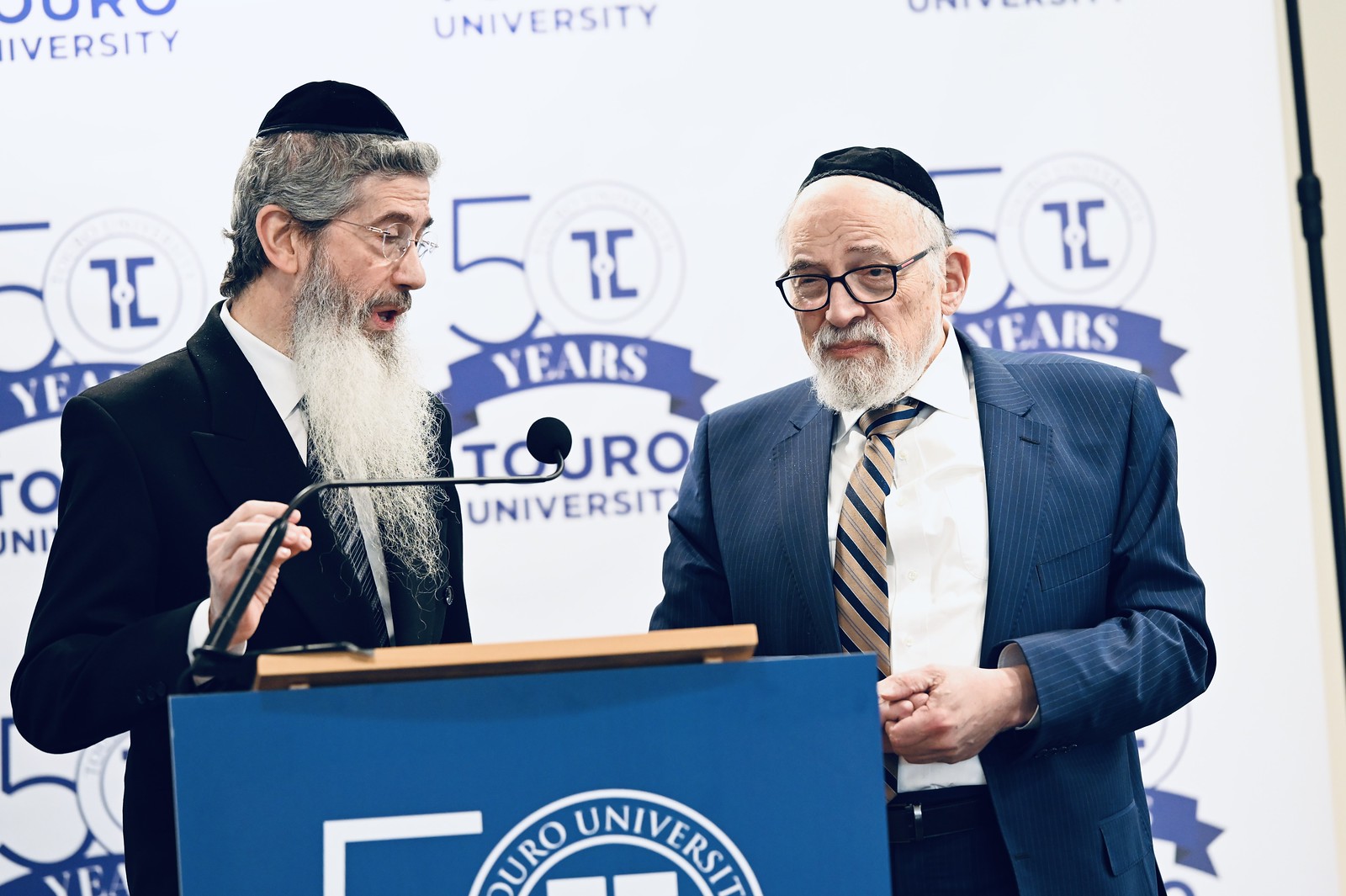The image depicts two older Jewish men standing behind a podium, which has a blue poster on it. Both men are wearing black yarmulkes. The man on the left has gray hair and a long gray beard and mustache, and he is dressed in a black suit with a white inner shirt and a tie. His hand is resting on a black microphone positioned on the podium, and he appears to be speaking. The man on the right is balding and has a much shorter beard. He is dressed in a blue blazer and a gold tie. In the background, there is a white backdrop with the words "50 Years Toro University" repeated in a pattern. The podium also features parts of the words "OURO" and "university" in blue. Both appear engaged in a discussion.